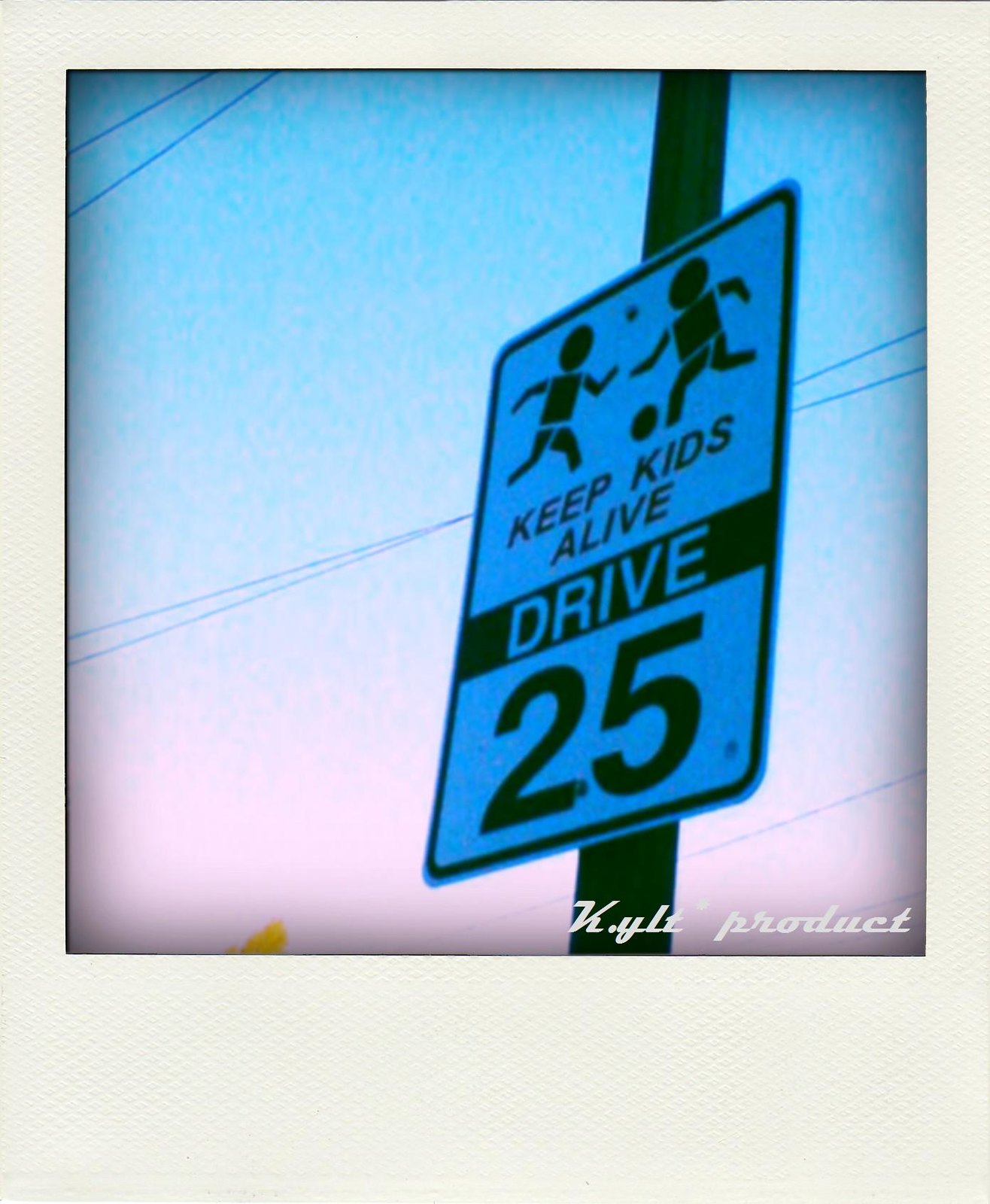The image features a stylized street sign, enhanced with a filter that lends a trendy pink and blue hue—blue at the top and pink at the bottom. The sign carries an important safety message, reading "Keep Kids Alive, Drive 25." The design on the sign includes simplistic, stick-figure-like illustrations of two children playing with a soccer ball, where one child is depicted kicking the ball to the other. The text is organized as follows: "Keep Kids Alive" at the top, followed by a black line with the white word "Drive," and then the number "25" on a white background with black text. The rectangular sign is mounted on a black pole. The white background of the scene features faintly visible telephone or electrical lines, suggesting the image was taken on a street.